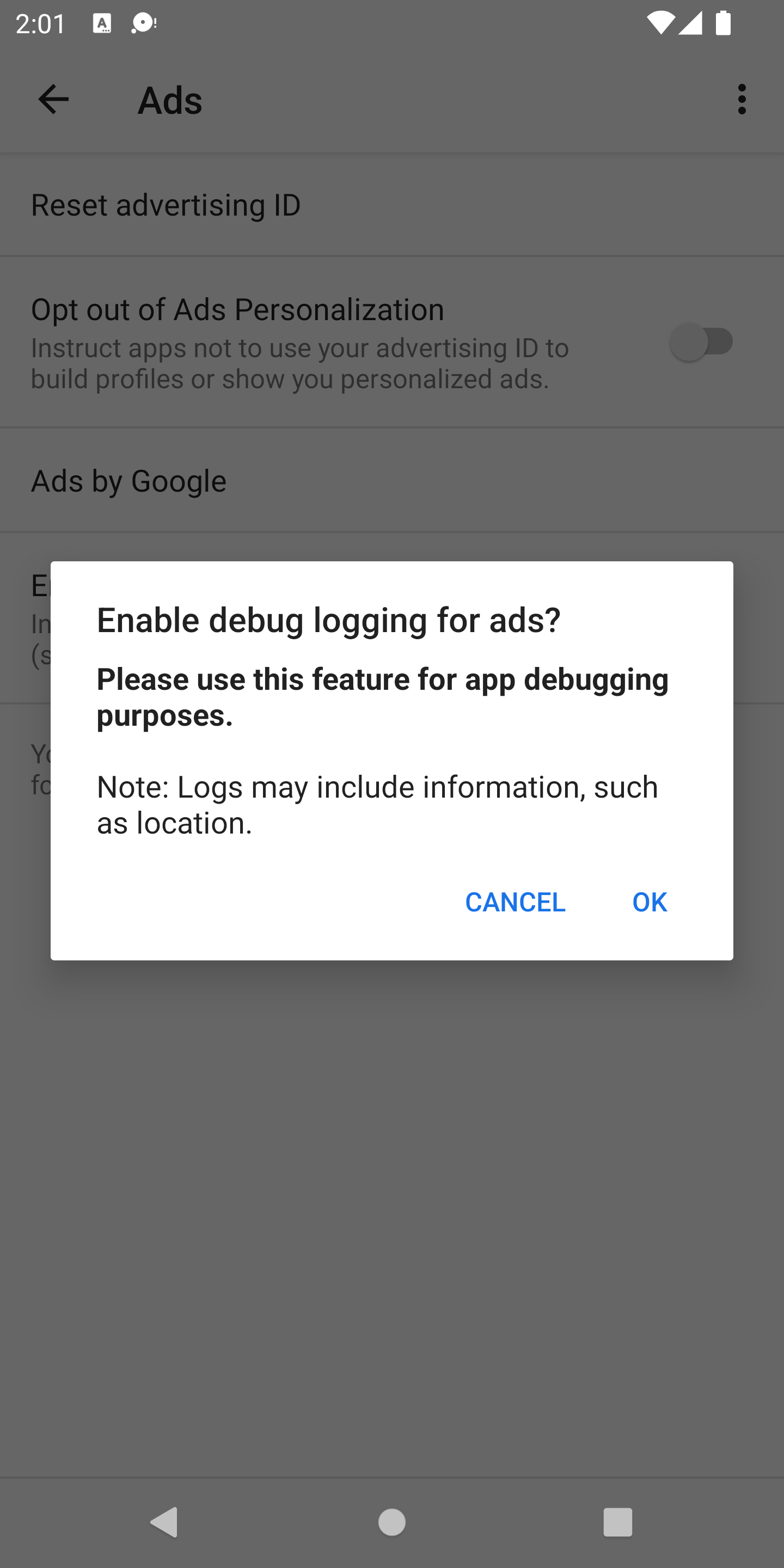A detailed caption for the image could be:

"A screenshot captured at 2:01 PM from an Android mobile device, displaying a partially obscured Ads settings screen. The interface shows the status bar at the top with a full Wi-Fi signal, cellular signal, and battery icons. A prominent white pop-up is centered on the screen, with the title 'Enable Debug Logging for Ads.' It advises using the feature for app debugging purposes and includes a note that logs may contain information such as location. Two options, 'Cancel' and 'OK,' are presented in blue at the bottom of the pop-up. The underlying Ads settings page is slightly visible, showing options like 'Reset advertising ID,' 'Opt out of Ads Personalization,' and 'Ads by Google,' with the rest of the options hidden by the pop-up."